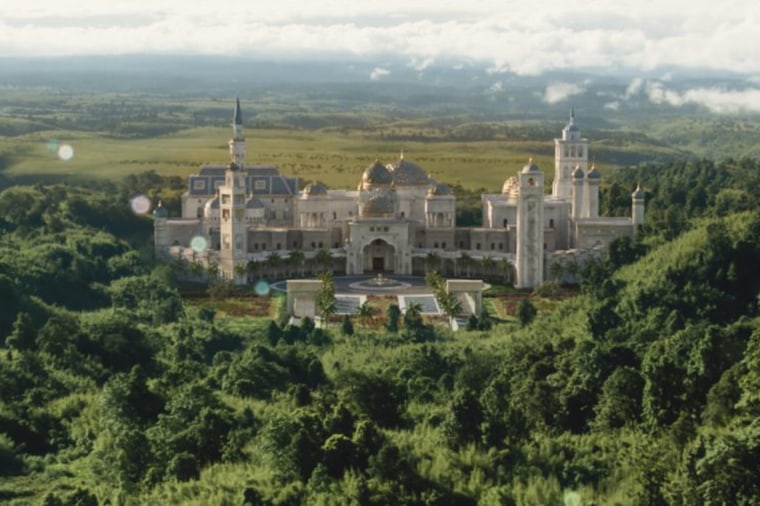This overhead view captures a sprawling castle nestled in the hills, surrounded by lush green vegetation, dense trees, and rolling hills on all sides. The castle, central to the image, is an expansive cream-colored structure trimmed in gold, featuring dark gray rooftops, two large domes, three smaller domes, several turrets, and three grand towers. In the front of the castle, two swimming pools and a large fountain can be seen amid the greenery. The land behind the castle stretches out into clear plains, with mountains and more greenery in the distance. The sky above is dotted with clouds, and the image also contains a few light flares on the left hand side. The overall scene is a vivid green landscape that seems distinctly rural and likely foreign, showcasing a magnificent and majestic architectural marvel at its heart.